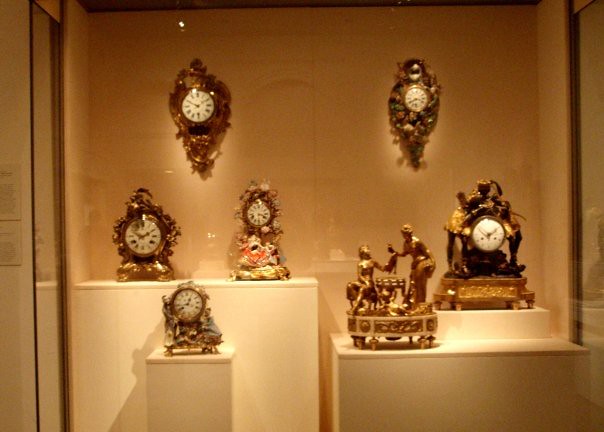This color snapshot captures an elaborate display of ornate golden clocks within a tall glass display case in a museum. The display features multiple clocks, with some mounted on the light beige back wall and others resting on white square or rectangular pedestals reminiscent of statue plinths. Each clock showcases intricate gold carvings around their faces, which are predominantly white, and include additional decorative elements such as human figures and colorful designs. One notable piece, situated at the forefront of the display, appears to be a musical clock or music box, intricately carved to depict a scene involving several people, possibly illustrating a mother and child. The entire arrangement, fully enclosed in the glass display, highlights the exquisite craftsmanship of these historical timepieces.